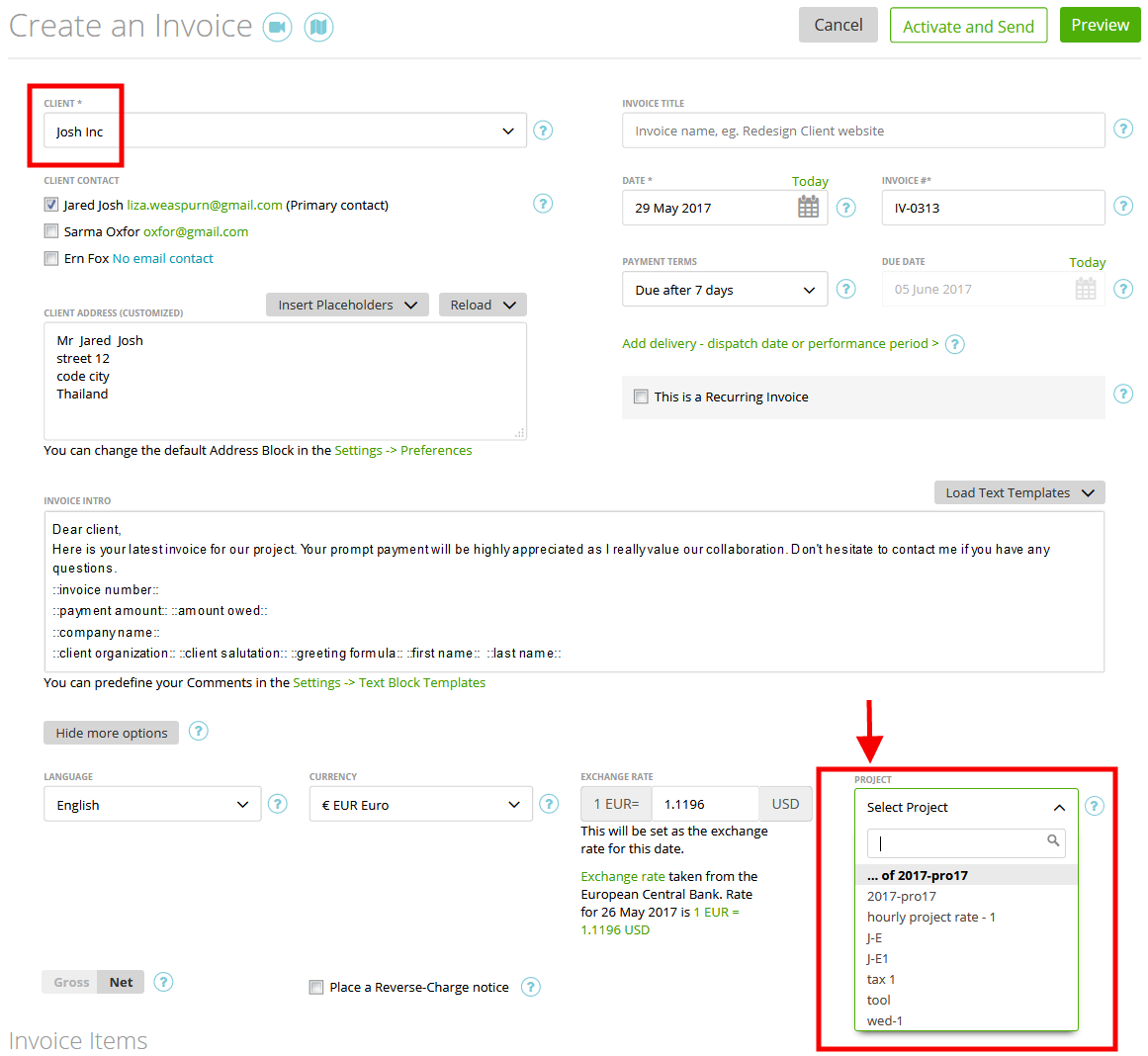A comprehensive invoice creation template is displayed in this image. At the top left corner, the title "Create an Invoice" is prominently labeled, accompanied by two small icons: one resembling a camera and the other a piece of paper. Adjacent to these icons, there are three actionable buttons: "Cancel," "Activate and Send," and "Preview."

Below the header, the template presents a detailed form designed to capture essential invoice details. The form includes sections for specifying the recipient, either a company or an individual, their address, and the date of invoice dispatch. Users can also select the method of sending the invoice and indicate whether the invoice is recurring or a one-time transaction. 

Furthermore, the template provides a text box for users to enter a personalized message to accompany the invoice. At the bottom of the template, there's a project assignment field, allowing users to categorize and save the invoice under a specific project for future reference. This highly versatile and user-friendly template found online is particularly crafted to streamline invoice creation.